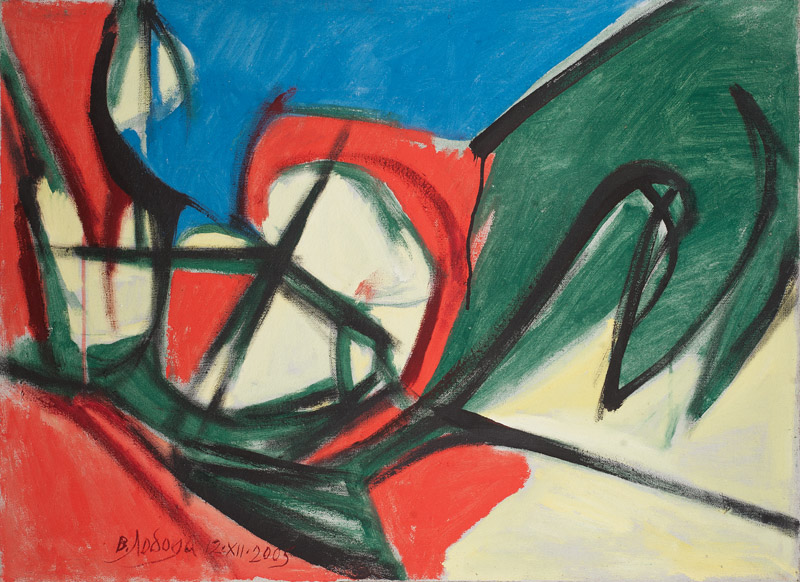An abstract painting, rendered in oils or possibly watercolor, showcases a dynamic array of colors and forms. The composition, wider than it is tall, features a multifaceted blue section at the top center. Dominant colors include black, white, gray, red, green, and blue, with noticeable elements like a black, curving line framing and intersecting various shapes. The painting's lower right-hand corner is primarily bright yellow with white, transitioning upward along a black line that branches out. A green line, undulating up to the upper right corner, contrasts against the blue on the upper left side, which features a blotch of red intersected by black and green stripes. The central area contains a red archway with green and black stripes, surrounding a white and yellow section. The left side blends red streaks intersected with blacks and greens, while the lower left corner is signed "B.A. DOGA" and dated 12 X 2 2003. This piece, reminiscent of a Rorschach painting, invites viewers to interpret its random shapes and vibrant splotches through their own perceptions.